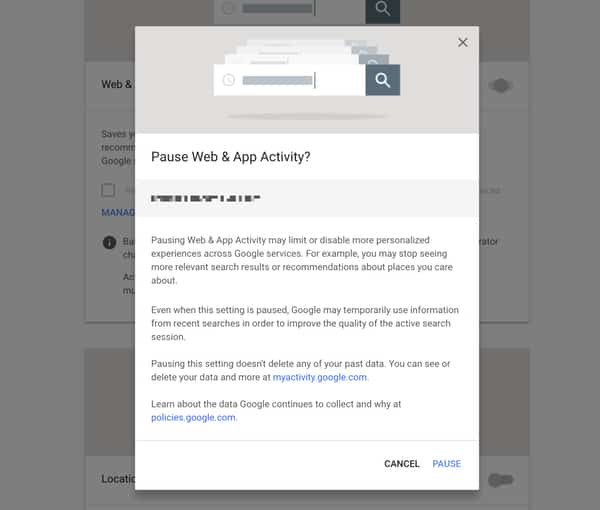This image is a screenshot of a webpage displaying a central pop-up box. The background of the page is grayed out, featuring a single column with various options, two of which are partially visible. Each entry begins with a beige header bar followed by a white section containing text. In the text, the top entry has "web" visible, but the rest is obscured by the pop-up box. Beneath the visible text in the top entry, there's a paragraph, a checkbox, a blue "Manage" link, and an information icon with a white "i," along with two bullet points. The bottom entry shows the beginning of the word "location."

The pop-up box itself is more vibrant in color, standing out from the grayed background. It also features a beige header at the top and displays a search bar with a clock icon, a gray horizontal bar, a vertical dividing line, and a dark gray or bluish square with a white magnifying glass on the right. This search bar appears repeated and fades backward, creating a visual effect of depth with each repetition growing narrower.

Below the search bar, there’s bold text stating "Pause web and app activity." Following this is a light gray rectangular section that resembles binary code or a graphical layout with rectangles and squares, almost like braille.

The main body of the pop-up contains three paragraphs of text. The text explains that pausing web activity may limit or disable more personalized experiences across Google services. For example, it may prevent users from seeing more relevant search results or receiving personalized recommendations about places they care about. Even when this setting is paused, Google might temporarily use information from recent searches to improve the quality of an active search session. Additionally, it clarifies that pausing the setting doesn’t delete any past data. It advises users that they can view or delete their data at the blue URL, "myactivity.google.com."

Further down, there's a line reading "Learn about the data Google continues to collect and why at," followed by the blue URL "policies.google.com."

At the bottom of the pop-up, beneath a dividing line, there are two action buttons: "Cancel" in black text and "Pause" in blue text, located in the bottom right corner.